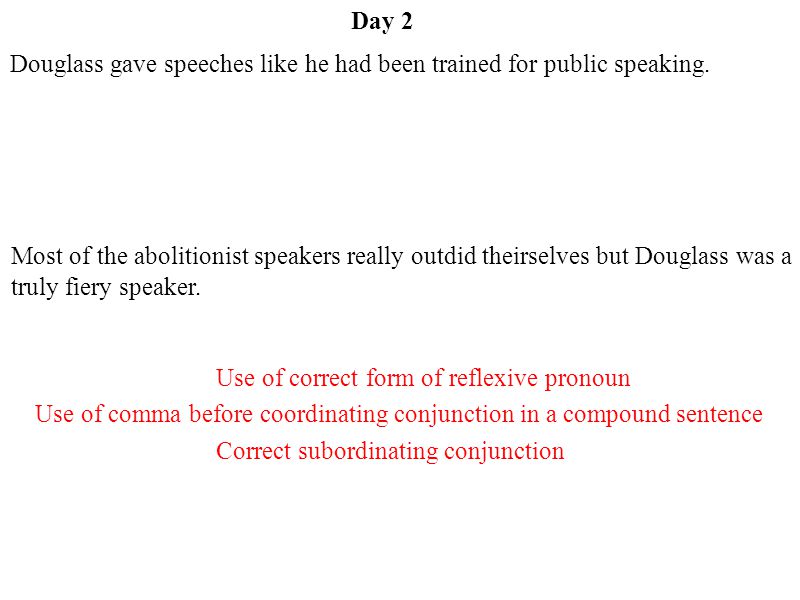The image features an excerpt from an English language textbook designed for students. Centered at the top of the page in bold text, it reads "Day 2." Below this, two sentences are presented in black: "Douglas gave speeches like he had been trained for public speaking." and "Most of the abolitionist speakers really outdid themselves, but Douglas was a truly fiery speaker." Directly beneath these sentences, instructions are provided in red text, which read: "Use of correct form of reflexive pronoun. Use of comma before coordinating conjunction in a compound sentence. Correct subordinating conjunction." These instructions suggest that students are expected to revise the sentences above by adding proper punctuation and making grammatical corrections.